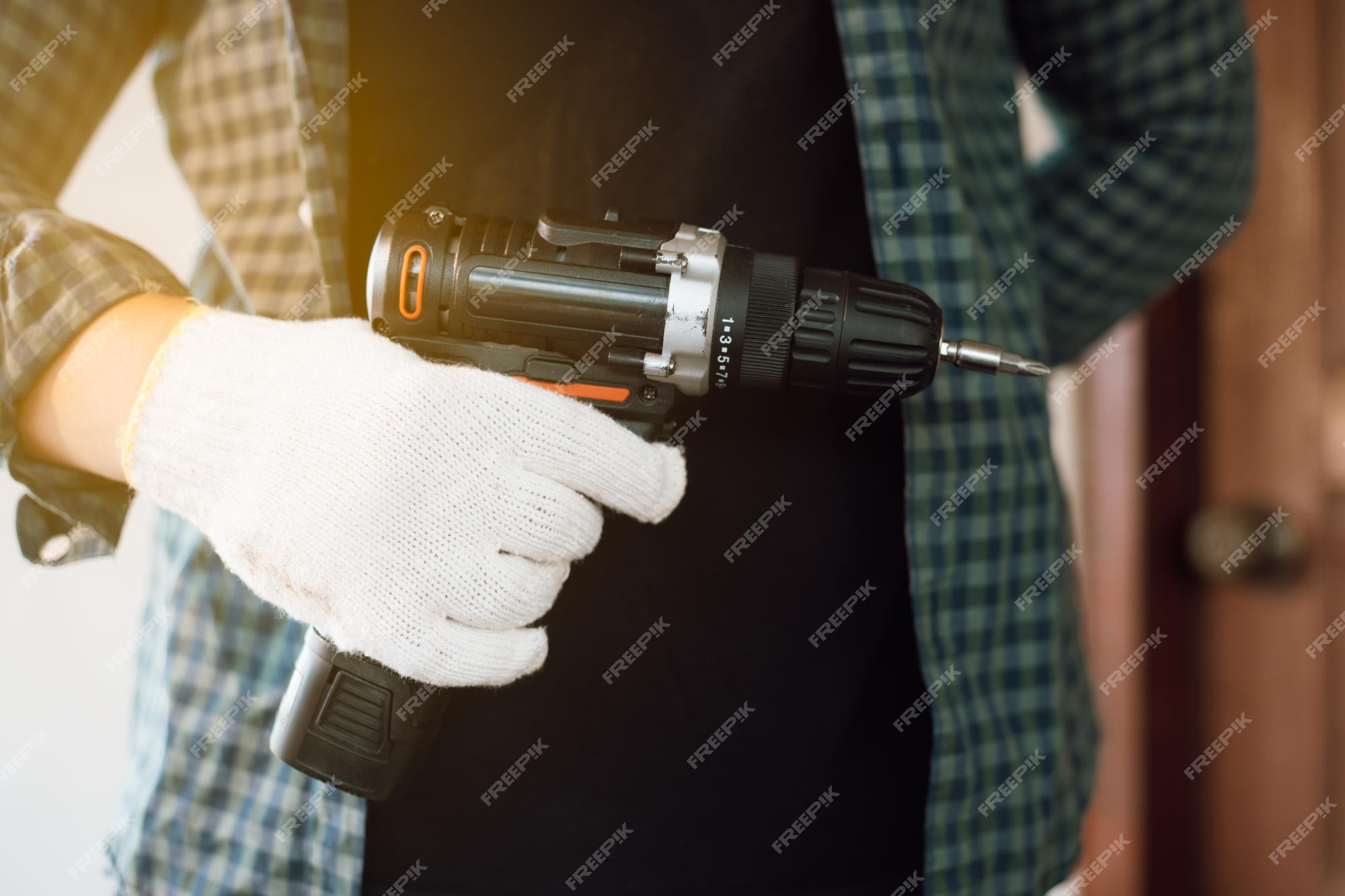The image depicts a person wearing a black shirt under an unbuttoned green and blue checkered long-sleeve shirt, standing front and center. Their right hand, clad in a white glove, holds a cordless black drill with orange and silver accents. The drill is oriented to the right, a Phillips drill bit attached. In the blurred background, a closed brown door with a doorknob is visible. The entire image is watermarked with the word "Freepik," diagonally ascending to the right. The lighting in the photograph suggests the time might be around sunrise.